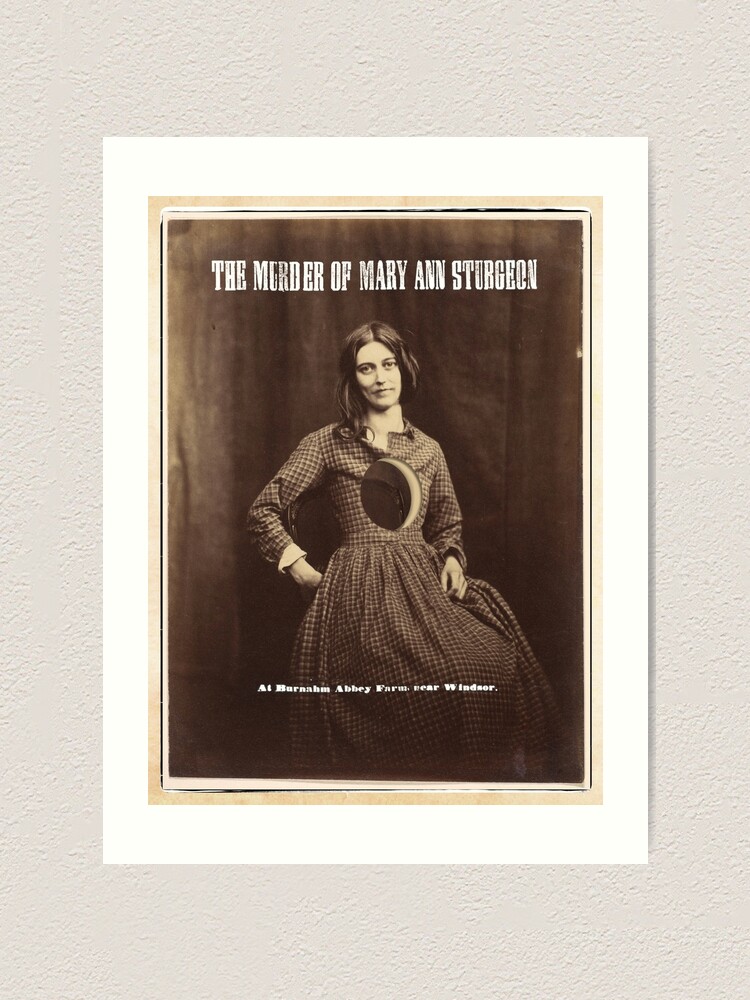The image depicts a sepia-toned photograph of a woman, framed within multiple borders: an outer gray border, an inner white border, and a thin tan border. The photograph appears old-fashioned, reminiscent of the late 1800s or early 1900s. The woman, likely Mary Ann Sturgeon as per the image's title, is dressed in an antiquated, long-sleeved dress adorned with dark dotted squares and white lines. Her arms are posed with a slight bend: her left arm forms a fist against her hip, while her right hand rests more loosely. Intriguingly, there is a conspicuous hole in the center of her chest area, revealing the brown background behind her. The title, "THE MURDER OF MARY ANN STURGEON," is emblazoned in capitalized white text at the top of the image. Below her, somewhat difficult to decipher, the text reads: "At Barnsham Abbey Warm Fear No Leader, at Barnham Abbey Farm Fear Windsor." This gives the impression of an old book cover or magazine, steeped in a narrative of historical intrigue.